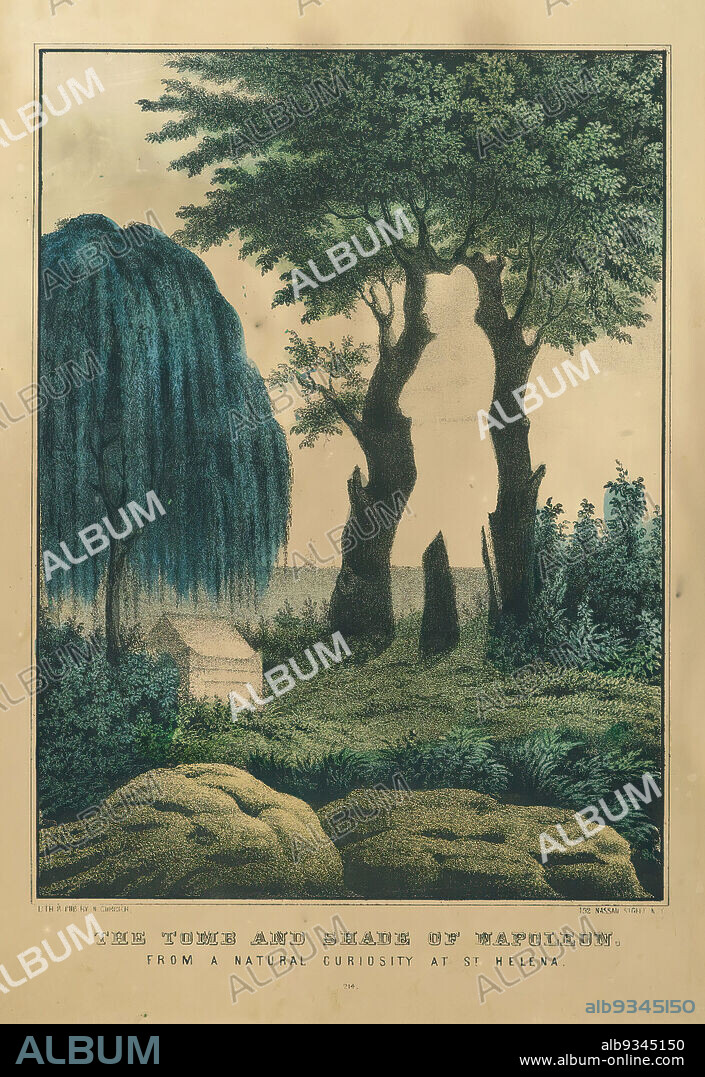The image is a detailed photograph presented as the cover of an old album titled "The Tomb and Shade of Napoleon Natural Curiosity at St. Helens," with a distinct diagonal watermark reading "Album." The cover features a vintage, finely drawn Chinese-style painting depicting a tranquil natural scene. On the left, there stands a weeping willow with dark aqua-blue leaves, offering a graceful, drooping silhouette. To the right, a pair of tree trunks merge into a single canopy of olive-colored leaves and branches. The background suggests a serene body of water, either a lake or a river, adding depth to the scene. A small white shed nestles near the right side of the weeping willow, subtly blending into the background. The foreground showcases lush greenery and vegetation along with large moss-covered rocks, enhancing the painting's sense of texture and natural beauty. The illustration is set on a light brown, slightly marbled piece of paper, further contributing to its vintage charm.